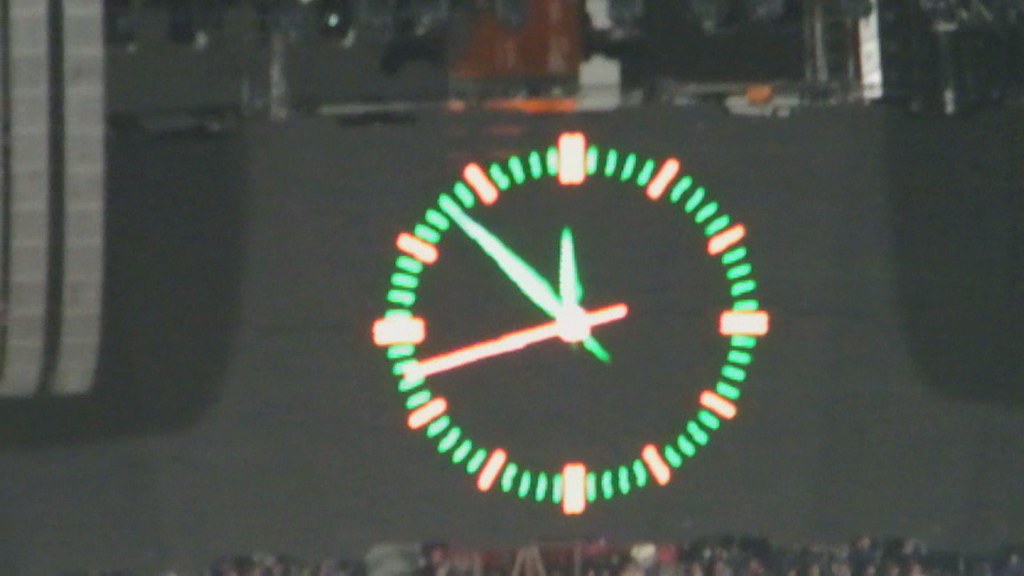This color photograph, displayed in landscape orientation, captures a slightly blurry close-up of a glowing digital clock inside what seems to be a sports arena. The clock, situated at the center on a gray background, features green minute marks and orange second marks, along with a green minute hand and an orange second hand, displaying the time at 11:53. Surrounding the clock are underlit objects, possibly machinery parts or architectural details, casting shadows. The lower portion of the image shows a crowd seated in bleachers, while the top portion hints at people sitting in what might be a booth, suggesting the setting of a sporting event under artificial lighting.